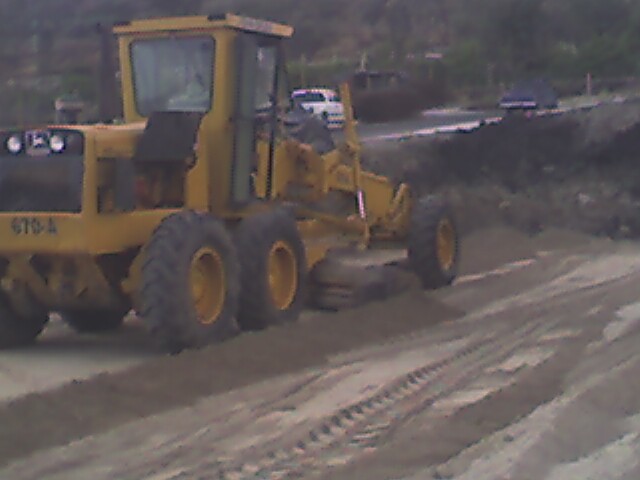A large, yellow truck with substantial black tires is traveling down a road that appears to be partially covered with snow or a similar substance. The skies are overcast, casting a dim light over the scene. Inside the cab of the truck, a driver is visible. In the background, opposite lanes of traffic can be seen with vehicles moving in the opposite direction. The overall ambiance suggests a chilly, possibly wintery day with the truck potentially being a snowplow in the process of clearing the road.